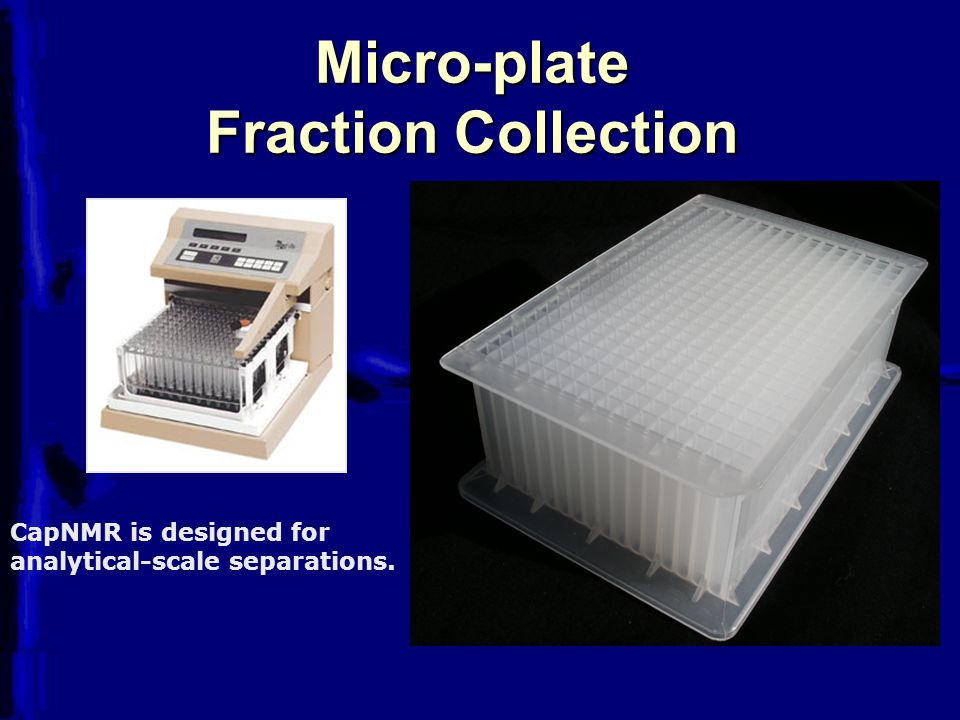The image is an advertisement, likely targeted at the medical industry, and it showcases the Microplate Fraction Collection system against a deep blue background. On the left side of the slide, positioned left-center, is the fully assembled product, which appears to be a machine with a tan-colored tray and a white base, designed for holding multiple test tubes. This tray features a keypad with approximately 10 to 12 keys. To the right, in a prominent separate image, there is a close-up of a clear or cloudy white plastic canister, situated on a black background, intended for holding the tubes during the separation process. The consistent text on the slide reads "Microplate Fraction Collection" in white lettering with a black outline at the top, and beneath the fully assembled product is the line "CAP NMR is designed for analytical scale separations," also in white lettering. The colors in the image prominently feature blue, white, tan, black, and clear elements, giving it an industrial and technical presentation style.